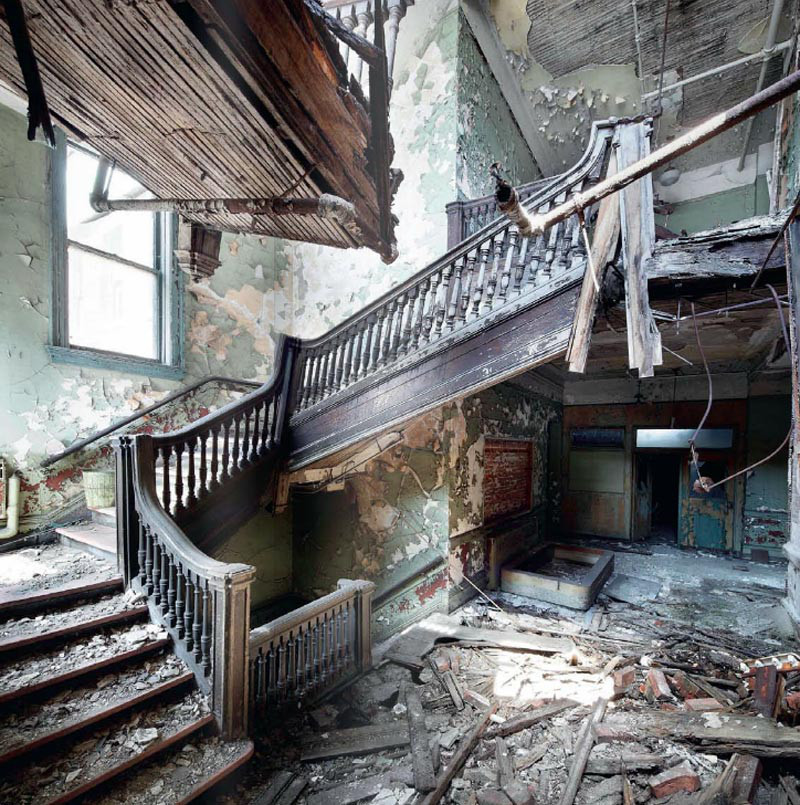The image shows the ruined interior of what once was an elaborate and possibly grand building, now completely condemned. A partially collapsed winding staircase with a wooden banister still stands, though most of the rails have fallen off. The staircase, leading up from the lower left to the upper right, indicates this might have been a multi-story structure, with sections of floors now entirely destroyed and debris scattered across the bottom floor. Sunlight streams through a large, intact window partway up the staircase, illuminating the decay. The walls, painted a peeling light green, add to the dilapidated vibe, suggesting the building might have been a hospital or hotel before its demolition. In the background on the right, a set of cracked wooden doors stands ajar, and a loose pipe dangles from the ceiling, disconnected. Despite the chaos and destruction, the basic outline of the structure remains intact, hinting at its former grandeur.